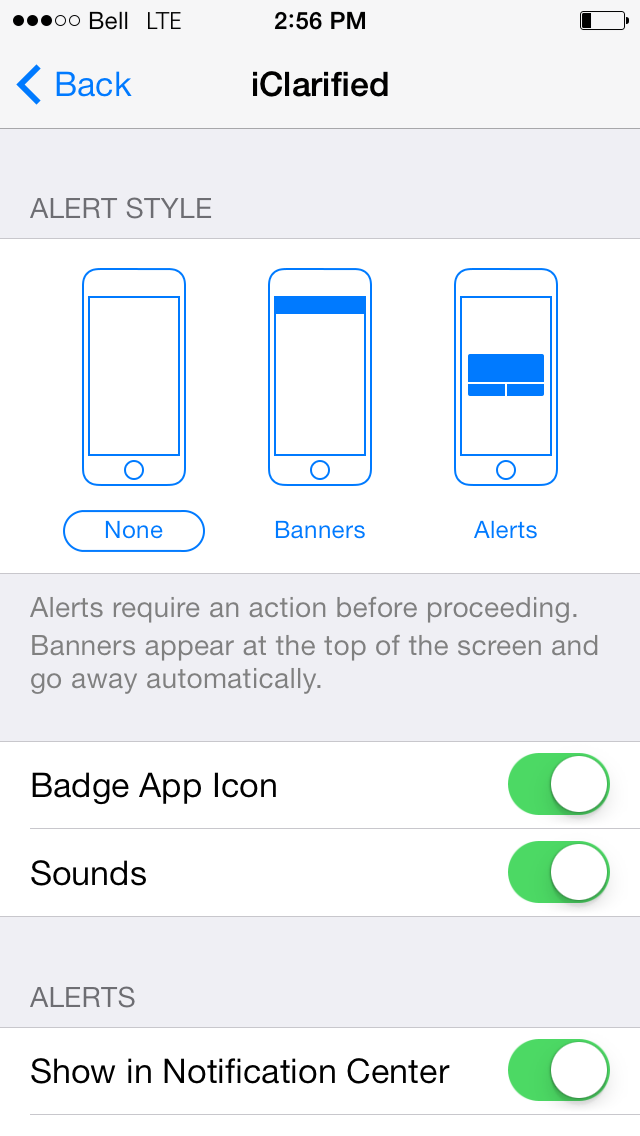This image is a screen capture from a cell phone displaying the interface of a notification settings menu within an application. At the very top of the screen, the status bar shows the company name of the cellular provider, the signal strength, the type of connection, the current time, and a battery strength meter on the right.

The interface is divided into several distinct sections. The topmost area is a gray navigation bar containing a back arrow labeled "Back" and the title of the current screen, which appears to be "Notifications."

Beneath this is a gray alert-style section. Directly below, occupying about a quarter of the screen's height, is a white background area displaying several notification settings options such as "None," "Banners," and "Alerts," each accompanied by a visual representation of how they appear on the screen.

Further down, another gray background bar provides a description: "Alerts require an action to be taken before proceeding. Banners appear at the top of the screen and go away automatically."

Additional notification settings follow, featuring several toggle switches for various choices:
- First is the "Badge App Icon" option, with the toggle switch slid to the right, indicating it is enabled.
- Below that is the "Sounds" option, similarly enabled with the toggle switch slid to the right.

This section is separated by another gray bar labeled "Alerts," beneath which is the "Show in Notification Center" option. This setting also includes a toggle switch, which is slid to the right and enabled.